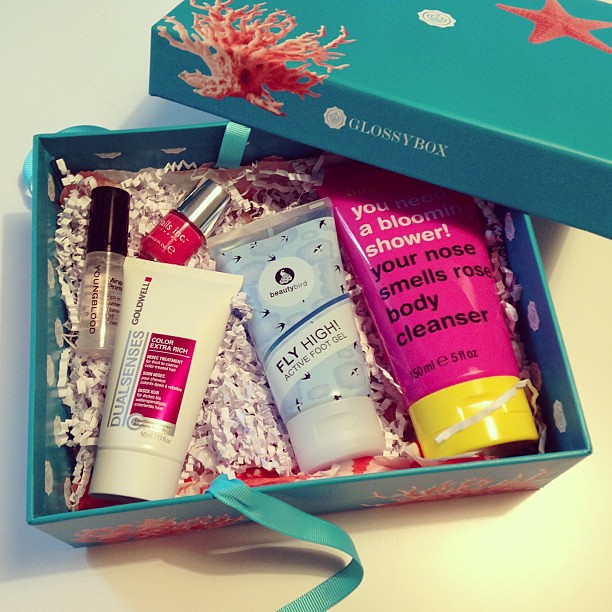This photograph features an open subscription box of beauty products, specifically from Glossy Box. The background showcases the lid, positioned in the top right corner, adorned with a pink starfish and coral design, and labeled with the brand name "Glossy Box" in white text. The box itself is a matching turquoise blue, and it contains five distinctive beauty items nestled in protective paper shavings.

Inside the box, there are three squeeze bottles and two smaller nail-related items. The most prominent item is a pink and yellow squeeze bottle labeled "You need a blooming shower, your nose smells rose body cleanser," indicating a floral-scented body wash. Next to it, a blue and white smaller bottle reads "Beauty Bird Fly High Active Foot Gel," a product designed for foot care. Adjacent to it is another white squeeze bottle labeled "Goldwell Dual Senses Color Extra Rich," hinting at hair care, specifically for color-treated hair.

Above these products is a small red nail polish bottle from Nails Inc, easily identified by its silver cap. Additionally, there is a clear bottle with a black cap labeled "Youngblood," which could be another nail product or possibly a nail polish remover. This thoughtful arrangement is cushioned by crepe paper, ensuring the products stay secure and protected in transit.